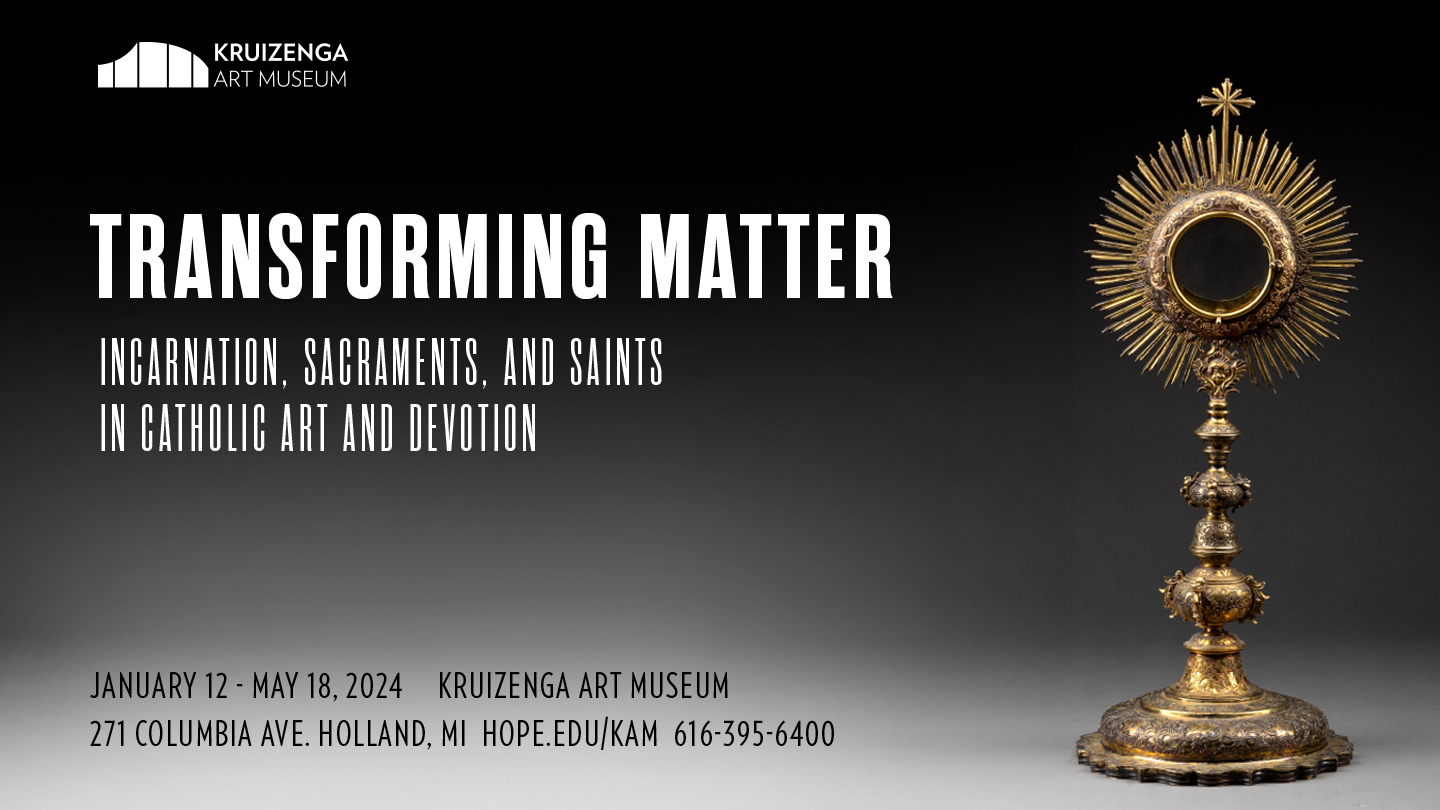This image, approximately two times as wide as it is tall, features a detailed promotional poster for an art exhibit titled "Transforming Matter: Incarnation, Sacraments, and Saints in Catholic Art and Devotion" at the Kruzenga Art Museum. The white text in the upper left corner includes the museum's logo followed by the exhibit title in larger font. Below, in smaller capitalized letters, it details the exhibition's theme. Further down, information in black text lists the exhibition dates as January 12th to May 18th, 2024, and provides the museum's address, 271 Columbia Avenue, Holland, Michigan, and contact information (hope.edu/kam and 616-395-6400).

On the right-hand side of the image, there is a detailed religious sculpture. This bronze-colored piece features a broad base from which a slender shaft extends upwards. Along this shaft, a series of round objects lead to an elaborate top section designed like a radiant sun with a hollow center encircled by spikes. At the very top, a cross with an X over it adds a finishing touch. The background of the image shifts from black at the top to light gray at the bottom, creating a contrasting backdrop for the text and sculpture.